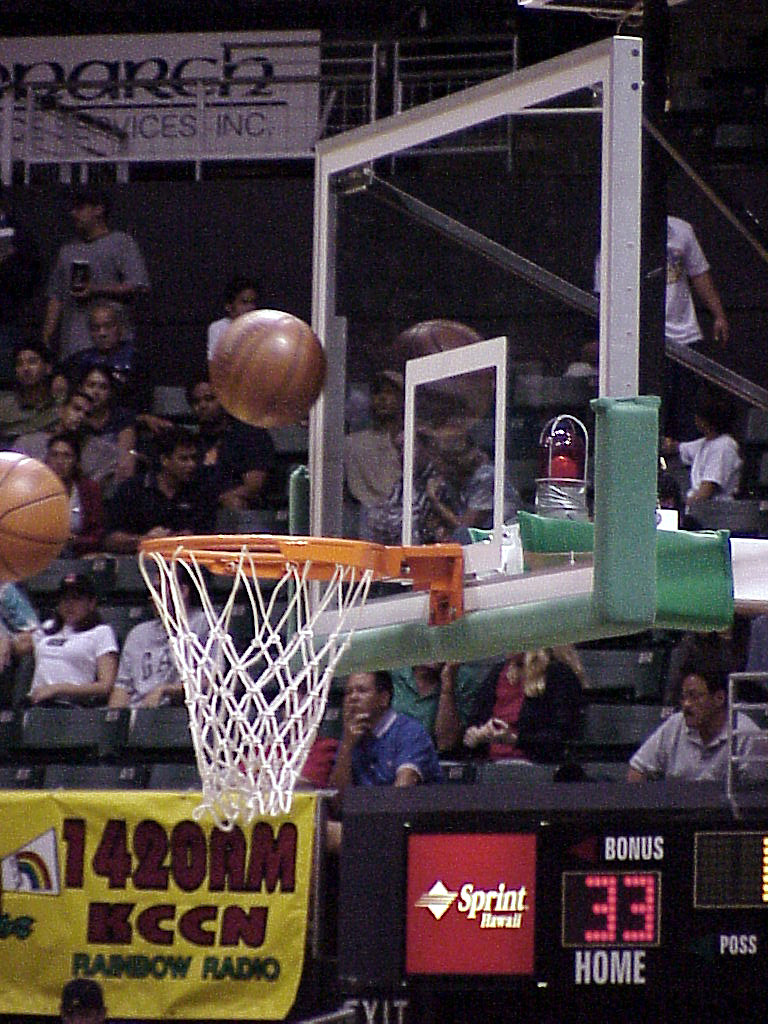This vivid image captures a moment in an indoor professional basketball stadium during what appears to be a warm-up before the game or at halftime. Dominating the scene is a clear backboard with a white square just above the orange metal rim, from which a white net hangs. The bottom of the backboard features a green base, and the entire apparatus is bordered with white lines. Two brownish-orange basketballs with black stripes are aimed at the hoop; one is hitting the backboard while the other is mid-flight.

In the foreground, a scoreboard displays "HOME 33 BONUS," suggesting a pause in the competitive action. Advertisements are clearly visible, including a Sprint sign on the left and a yellow banner for 1420 AM KCCN Rainbow Radio. Behind the hoop, the seating sections are mostly occupied, with spectators intently watching something happening to the left of the frame. This engaging scene captures the anticipation and excitement of the game, with every detail highlighting the energetic atmosphere of the basketball arena.